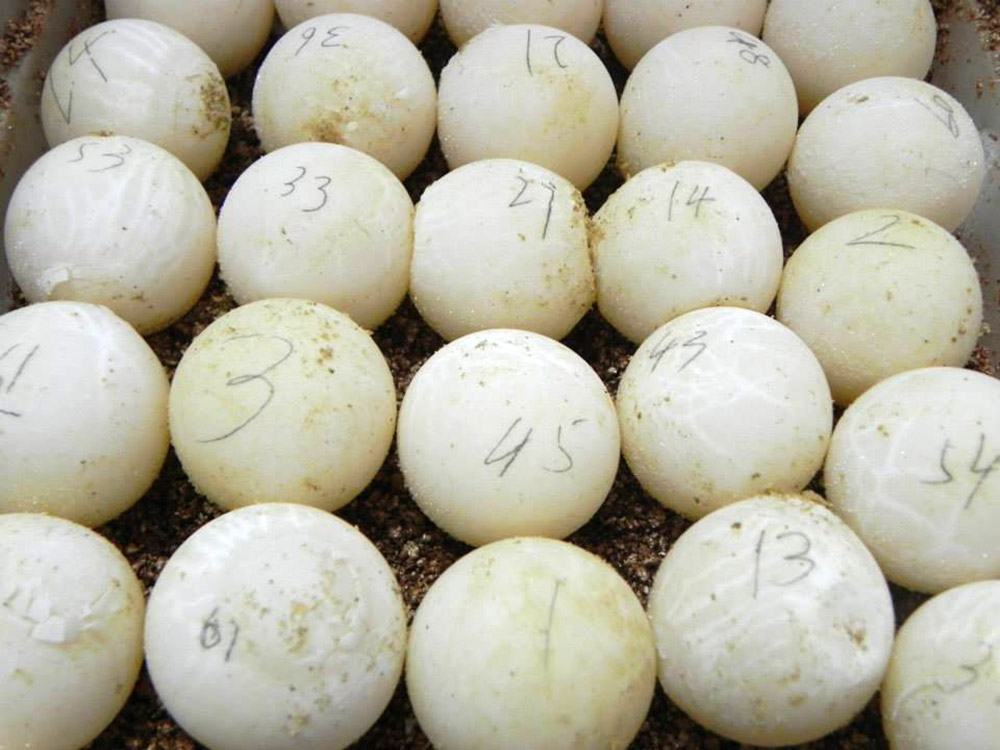The image depicts 25 off-white spherical objects, arranged meticulously in 5 rows of 5, nestled in a dirt-filled setting. They are primarily identified as eggs, possibly turtle eggs, though there is some ambiguity with some observers mistaking them for ping-pong balls. Each egg is marked with a different number, written in pencil. The visible numbers vary widely, including 1, 2, 3, 13, 14, 18, 21, 24, 27, 33, 36, 43, 45, 48, 53, and 61. The eggs are about the size of tennis balls, with one in the lower left corner showing signs of cracking or peeling. The eggs are quite aged and dirty, further blending in with the earthy surroundings of the crate or box they are housed in. Despite the randomness of the numbering, the organized rows and worn condition of the eggs create a strikingly detailed and intriguing scene.